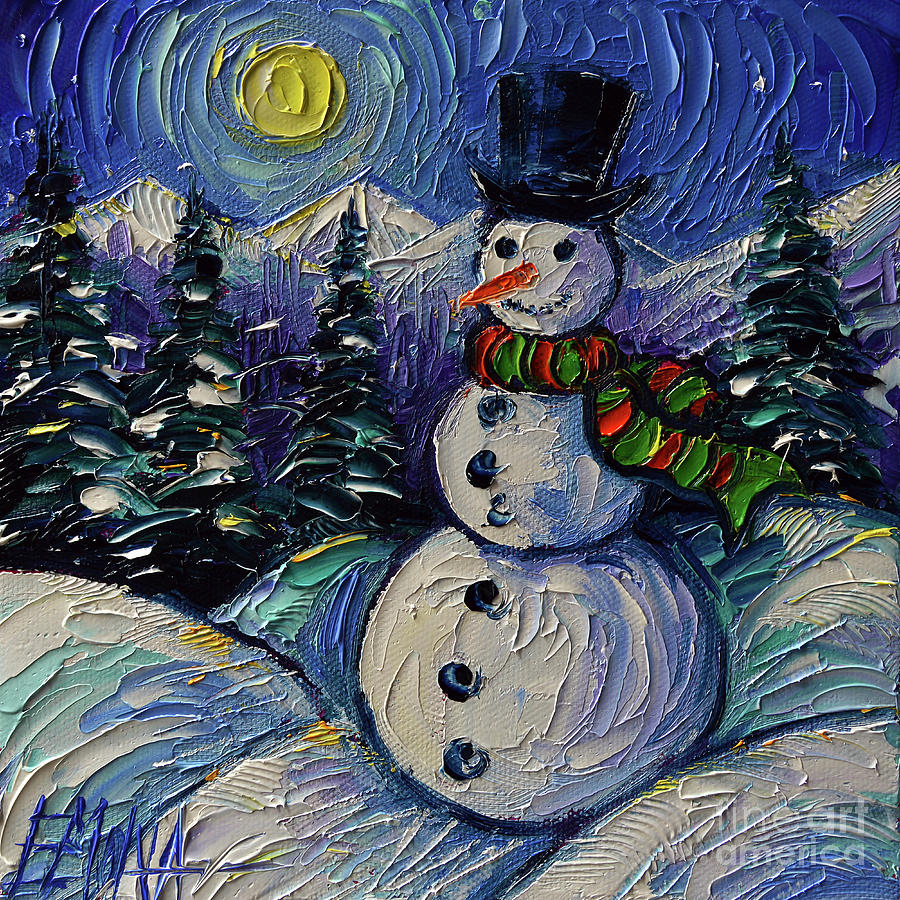The image depicts a textured painting of a snowman in a snowy landscape, likely created using a palette knife to achieve a raised texture. The scene is illuminated by a bright yellow sun set against a vivid blue sky. Below the sun, its reflection shimmers on a series of snow-covered mountains that span the background. Nestled among the mountains are four pine trees—three on the left and one on the right—painted in dark green hues with snow clinging to their branches. 

Dominating the foreground, a jolly snowman sits slightly to the right of center, composed of three snowballs stacked with a large lower body, a smaller mid-section, and a round head. The snowman is adorned with a black top hat, a red and green striped scarf, a carrot nose, two round eyes, and a smiling face. Six black buttons run vertically down its body. The snow beneath the snowman includes touches of white, light blue, blue, and yellow, adding depth and variation in color.

Both the left and right bottom corners of the painting bear inscriptions: the left side has a blue signature, which is illegible, and the right side features a watermark reading “Fine Art America.” The scene captures a bright and clear winter day, beautifully detailed and inviting.